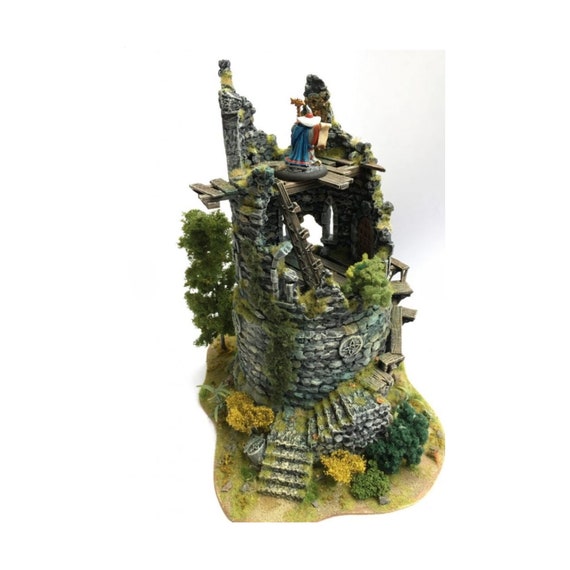This is an intricate photograph of a porcelain or ceramic sculpture, potentially a child's playset, depicting an ancient stone tower in ruins. The structure stands on a base adorned with scattered brown dirt, lush green shrubs, and several diminutive trees. At the front of the sculpture, there are cement steps that ascend directly to a partial structure before winding to the right. The stone tower, visibly weathered and worn, is covered in patches of green moss, giving it a rustic and aged appearance. The ruins show signs of disrepair and damage, suggesting that the tower was once part of a larger building, possibly a castle, that has since fallen apart. At the very top of the tower, a lone figure stands on what appears to be wooden panels. This figure is dressed in a blue or green robe with white accents around the neck, observing the scene below. The detailed and verdant scenery combined with the worn architecture paints a vivid picture of a storied past, blending elements of history, decay, and nature's reclamation.